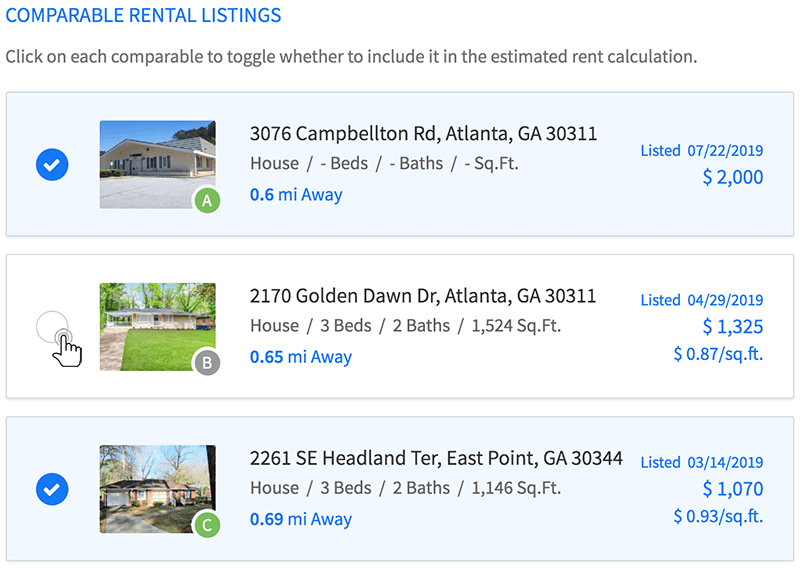This image captures a user interface from a real estate application or website, though the specific platform is unidentified due to the absence of a URL or other distinctive markings. At the top, the title "Comparable Rental Listings" is prominently displayed in blue font against a clean, white background. Below this, a gray font instructs users to "click on each comparable to toggle whether to include it in the estimated rent calculation."

The interface is divided into three distinct sections or boxes. The first box, with a light blue background, features a blue check mark on the left. Next to this check mark is an image of the property, followed by its address. The box includes fields for the number of bedrooms, bathrooms, and square footage. Additionally, information is provided in blue font about the property's distance in miles, its listing date, and cost, which are aligned to the right.

The second box stands out with its white background and a thin gray outline. It shows a pointer finger icon, suggesting user interaction to select the property by checking the circle, which turns blue upon selection. Similar to the first box, it contains a property image, address, number of bedrooms, bathrooms, square footage, distance, listing date, cost, and uniquely, the cost per square foot.

The third box, labeled as "House C," also has a blue background, indicating it is selected. It includes the same detailed information as the previous boxes: property image, address, number of bedrooms, bathrooms, square footage, distance, listing date, cost, and the cost per square foot.

Overall, this interface provides a comprehensive, user-friendly layout for comparing rental property listings, complete with all necessary details for making informed decisions.